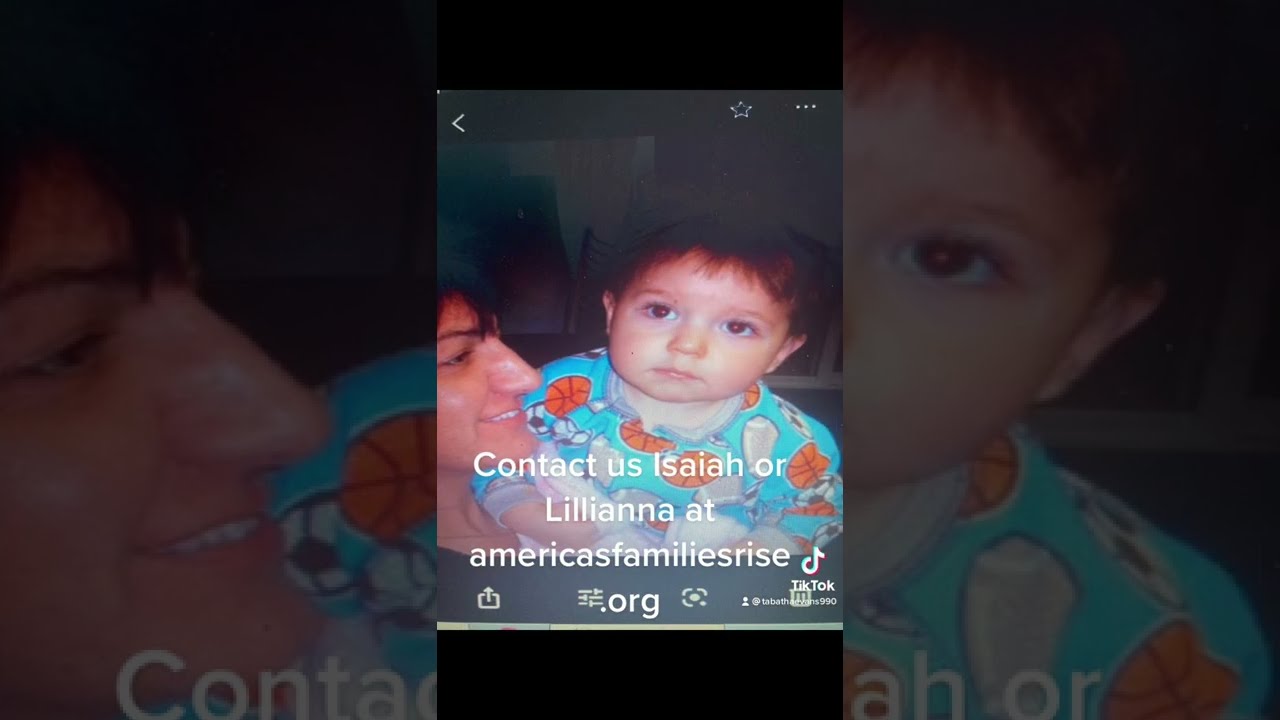The image is a screenshot from a TikTok video. It features a young child held by an adult woman, both with darker complexions and short dark hair. She is smiling and facing to the right, showing only half of her face. The child, wearing blue pajamas patterned with basketballs and soccer balls, has brown hair and big brown eyes and is looking slightly off-center towards the camera with a neutral expression. Behind the central image, there's a zoomed-in, faded version of the same picture, creating a border effect with black strips on the top and bottom edges. Text overlaying the image reads, "Contact Us, ISAIAH, ISAIAH, or LILLIANA at AmericasFamiliesRise.org" in four lines. The TikTok logo is also visible in the bottom right corner. Additional interface elements include a star, three dots for more options, a left arrow, and various buttons.